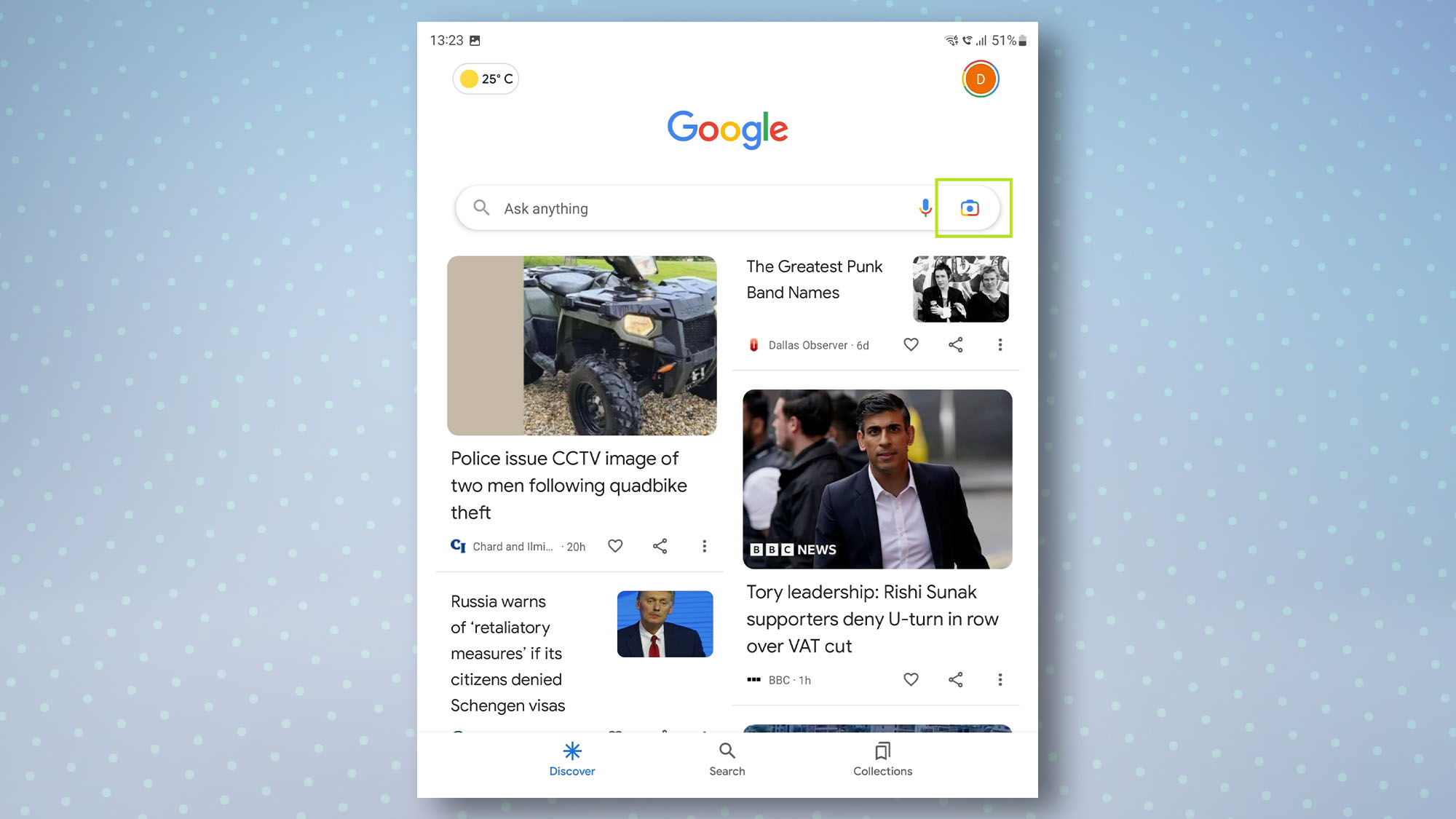The image features a Google search page with an overlay against a two-toned light blue background. The upper half of the background is a slightly darker blue, transitioning to a lighter blue towards the bottom, and is scattered with tiny light blue dots. 

At the top center of the Google page, the time is displayed in military format as 13:23, with a small icon adjacent to it. On the right-hand side, there are several icons: one resembling a phone, another indicating signal strength, a battery icon that appears to be at 51% capacity, and lastly, a battery icon that is halfway full. Below these, there is an orange circle featuring the letter "D," bordered with a different color. 

On the left-hand side, the temperature reads 25 degrees Celsius accompanied by a sun icon. Dominating the middle of the screen is the Google logo in its iconic rainbow colors. Beneath the logo, there is an oval-shaped search bar that reads "Ask Anything" with a microphone icon on the right side and a camera icon outlined in green to the left.

On the main section of the webpage, there are media images and articles available for viewing. One highlighted article is titled "Police Issue CCTV Image of Two Men Following Quad Bike Thefts," alongside other articles, each featuring accompanying images, share buttons, and favorite buttons.